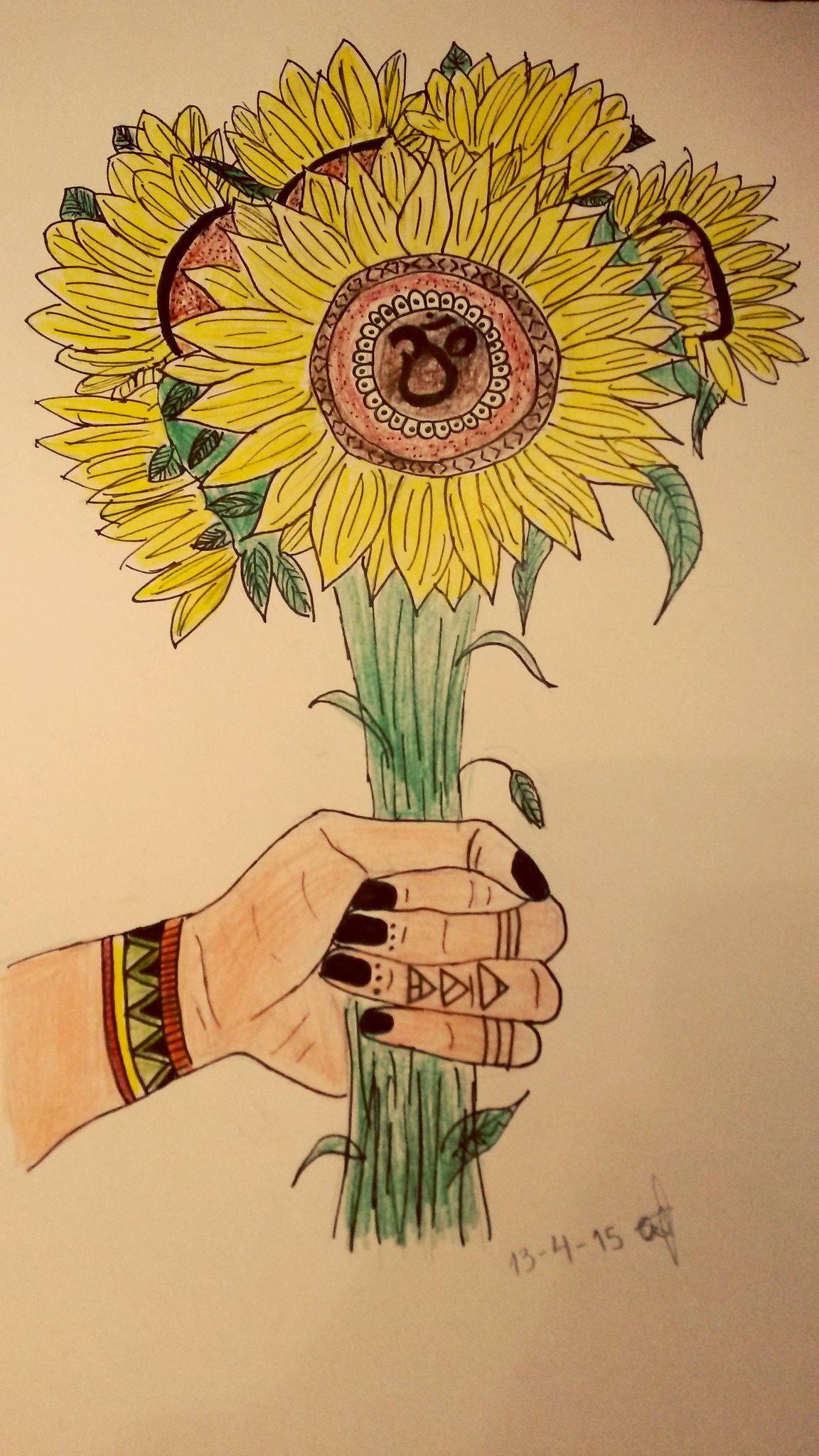The rectangular color drawing, oriented vertically, features a detailed depiction of a white hand emerging from the lower left corner. The hand is adorned with a bracelet that bears a design reminiscent of Native American Indian patterns. The fingers of the hand are delicately wrapped around several green sunflower stalks, which extend upwards through the hand. At the top of these stalks, numerous sunflower blossoms burst into view, their vibrant yellow petals radiating in various directions, though the exact number is not discernible. The fingernails of the hand are painted black, and the second finger from the bottom showcases three small, rectangular tattoos. In the lower right corner of the drawing, the date "13415" is inscribed in a scribbly font.